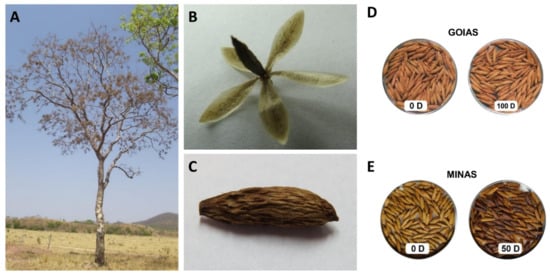This composite image consists of five distinct photos labeled A through E. 

- **Photo A:** Depicts a tree with sparse foliage situated in a grassy field, possibly during the fall. The background features yellow grass and some hills, and to the right edge, another tree with greener leaves is partially visible.
  
- **Photo B:** Shows a flower or plant with five to six leaves arranged in a star pattern on a white surface.
  
- **Photo C:** Displays a rough-textured brown seed or nut placed on a white surface.
  
- **Photo D:** Is labeled "Goyas" and contains two small circular dishes filled with long, rice kernel-like seeds. The first dish is labeled "0D" and the second "100D," with the seeds appearing orange in color.
  
- **Photo E:** Labeled "Minas," it also includes two circular dishes, but of darker seeds compared to photo D. The first dish is labeled "0D" and contains yellow seeds, while the second, labeled "50D," contains brownish seeds.

This detailed arrangement highlights various natural elements and comparisons of seed types.